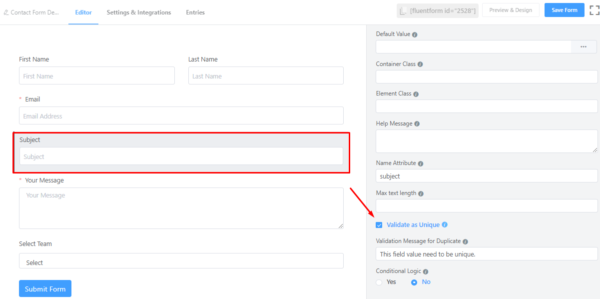This screenshot depicts an online form editor interface, specifically a "Contact Form" with various settings and fields for customization. In the upper left-hand corner, the navigation menu includes tabs labeled "Contact Form," "Editor," "Subscriber Settings," "Integrations," and "Entries." The "Editor" tab is highlighted in blue, indicating it is the currently active section.

Within the active "Editor" interface, several form fields are presented for user input. These include:
- "First Name" with an accompanying text box
- "Last Name" with an adjacent text box
- "Email" labeled as a required field, signified by an asterisk, with a text box below it
- "Subject," which is encapsulated within a red rectangle, highlighting its significance. An arrow points from "Subject" to a "Validate as Unique" checkbox
- "Your Message" marked as a required field
- "Select Team" with a dropdown selection labeled "Select"

At the bottom of the form, there is a prominent blue "Submit Form" button with white text.

On the right-hand side of the screen, additional settings are available for further customization of the form fields. These settings include:
- "Save Form" and "Preview" options in the upper right-hand corner
- Beneath these, various attributes and options such as "Default Value," "Container Class," "Element Class," "Help Message," "Name Attribute," "Max Text Length," and "Validate Message for Duplicate," with corresponding text boxes for input
- An option for conditional logic, presented as a toggle between "Yes" or "No"

This detailed editor interface allows users to meticulously configure the contact form's appearance and functionality, ensuring a tailored experience for form submissions.